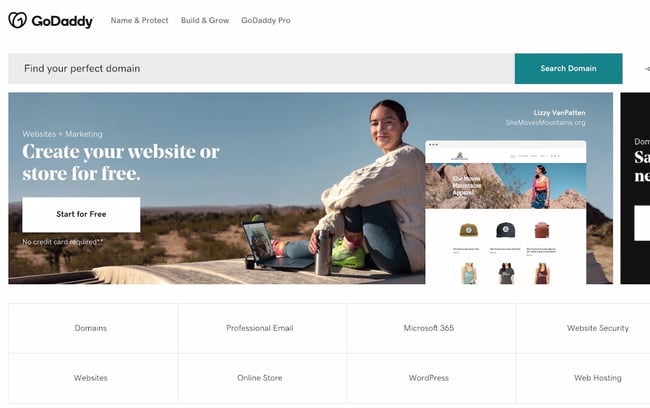Here is a detailed, cleaned-up caption for the described image of the GoDaddy landing page:

---

The landing page screenshot for GoDaddy prominently features their new logo in the top left-hand corner, resembling a heart turned sideways. Adjacent to this logo, bold black text spells out "GoDaddy" with capitalized "G" and "D."

Below the logo, three clickable buttons in standard black text read: "Name and Protocol," "Build and Grow," and "GoDaddy Pro."

In the center of the page, within a dark gray and black rectangle, the headline "Find Your Perfect Domain" is displayed.

To the right of this section, there's a clickable teal button with white text that reads "Search Domain."

Just below, a large rectangle features an image of an Asian woman sitting with her knees drawn to her chest. She dons neon green shoes, blue jeans, and a long flannel shirt colored white with streaks of peach or off-gray. A black laptop with an active screen is placed nearby. Surrounding her are a few items, including a close-up of a web page that resembles a Mac interface, indicated by the three iconic circles in the top left corner.

On the right-hand side of the image, there is a woman in a short-sleeved red shirt and blue shorts. She has shoulder-length black hair. Next to her, some white text is visible but difficult to read due to blurriness. Nearby, there are two hats—one tan and one black—and another brown item.

Additionally, three women, whose heads are mostly out of the frame, are pictured. They are wearing tank tops in gray, black, and maroon or brown.

Toward the top-right corner, the name "Lizzy Van Patten" is displayed, along with her website "SheMovesMountains.org," capitalizing the initials S, M, and M. 

On the left-hand side, more white text reads "Websites + Marketing." Below it, in bold white text, "Create Your Website or Store for Free" is prominently shown, followed by a clickable white button with black text that says "Start for Free." Underneath this, additional white text states, "No Credit Card Required" with an asterisk symbol indicating terms or conditions apply.

---

This captures the structured, detailed elements of the GoDaddy landing page as described.